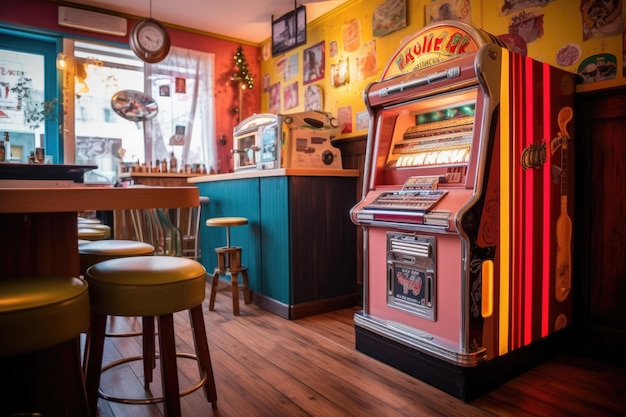The image portrays a rendered scene of an old-fashioned diner prominently featuring an antique jukebox on the right side. The jukebox, reminiscent of an arcade machine, has a dome-shaped top with red letters spelling "ROLL" and a design suggesting roller skates or dancing shoes. Its color scheme combines shades of pink, yellow, and brown, with chrome accents around its bulky body, further accentuating its vintage allure. The jukebox is positioned against a wall that is paneled halfway up with wood, transitioning into bright mustard yellow adorned with various signs and pictures.

To the left of the jukebox, there is a teal-colored diner counter equipped with an old-school metallic register and a classic soda fountain. Yellow stools with brown wooden legs line the counter, and a separate table is visible towards the establishment's blue-colored door. In the background, a blue counter with more stools stands in front of a front window, near which hangs a round clock. The room's decor also features hardwood flooring and a combination of yellow and red on the walls, adding to the nostalgic atmosphere. The overall scene is devoid of patrons and bathed in daylight, with an inviting glimpse of the outside.